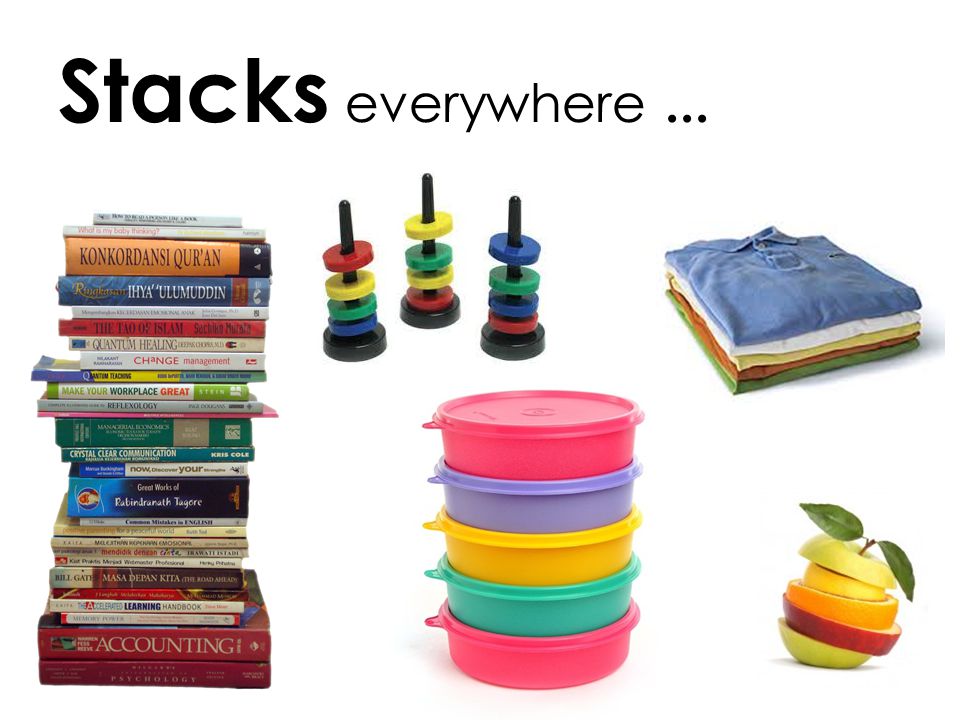The image presents a diverse assortment of stacked items against a white background, summarized by the title at the top, "Stacks Everywhere...". On the left side, there's a tall stack of approximately 15 books, including titles such as "Kandor Danzig" and "Accounting", the latter distinguished by its red cover. In the central portion of the image, three rod toys display four wings each in red, yellow, green, and blue. Below these are five stacks of Tupperware containers in colors pink, turquoise, yellow, and green, with the top container featuring a lid. On the top right, a neat stack of men's polo shirts in blue, white, yellow, orange, and green is visible. Finally, at the bottom right, neatly sliced fruits are stacked, featuring apple slices, lemon slices, orange slices, and slices of different-colored apples. The varied colors and positions of these objects suggest an educational or presentation setting.